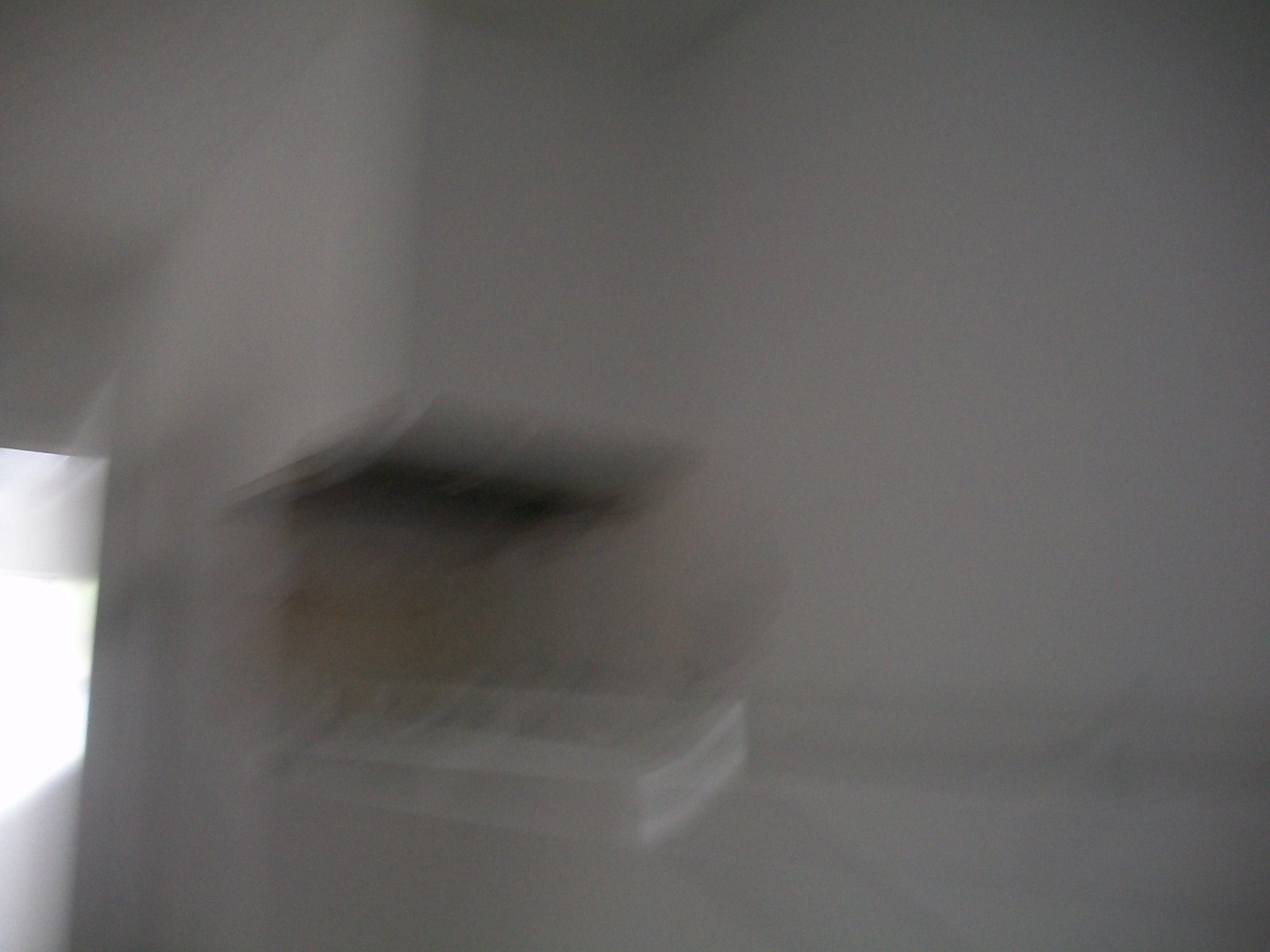The photograph captures a scene in a dimly lit room or hallway and is noticeably blurred, indicating motion either from the camera or the subject. In the bottom left corner, there is a faint outline of a doorway, suggesting an indoor setting. The right side of the image features a wall that appears light grey due to the low lighting, though it could actually be painted white. Near the center bottom of the photo, there is an indistinct opening with a grid pattern, possibly an air vent or part of a ventilation system. A rectangular white shape towards the bottom middle of the image, distorted by the blur, might be a control panel or switches, likely related to the air conditioning or heating system. The overall effect of the blurred photograph suggests a streaked, elongated appearance of any identifiable objects, making the precise identification challenging but hinting at typical indoor fixtures.